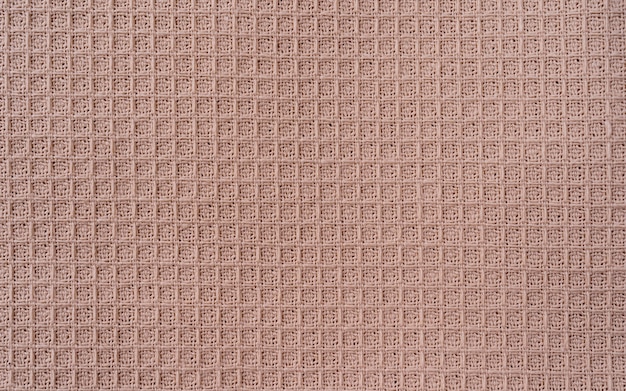The photograph presents an extreme close-up view of a piece of fabric, prominently displaying a pattern consisting of dozens of meticulously arranged small squares. This pinkish or rose-colored material could be typically found in items that require detailed work such as bandages or possibly a woven blanket or sheet. The image captures only the fabric, with no other objects visible. Each small square is bordered by vertical and horizontal stitching, contributing to a textured appearance. In addition, some squares feature tiny oval-shaped stitching with minute holes, adding to the intricate detail of the fabric. The photograph is taken with high clarity and bright lighting, emphasizing the fabric's texture and color.